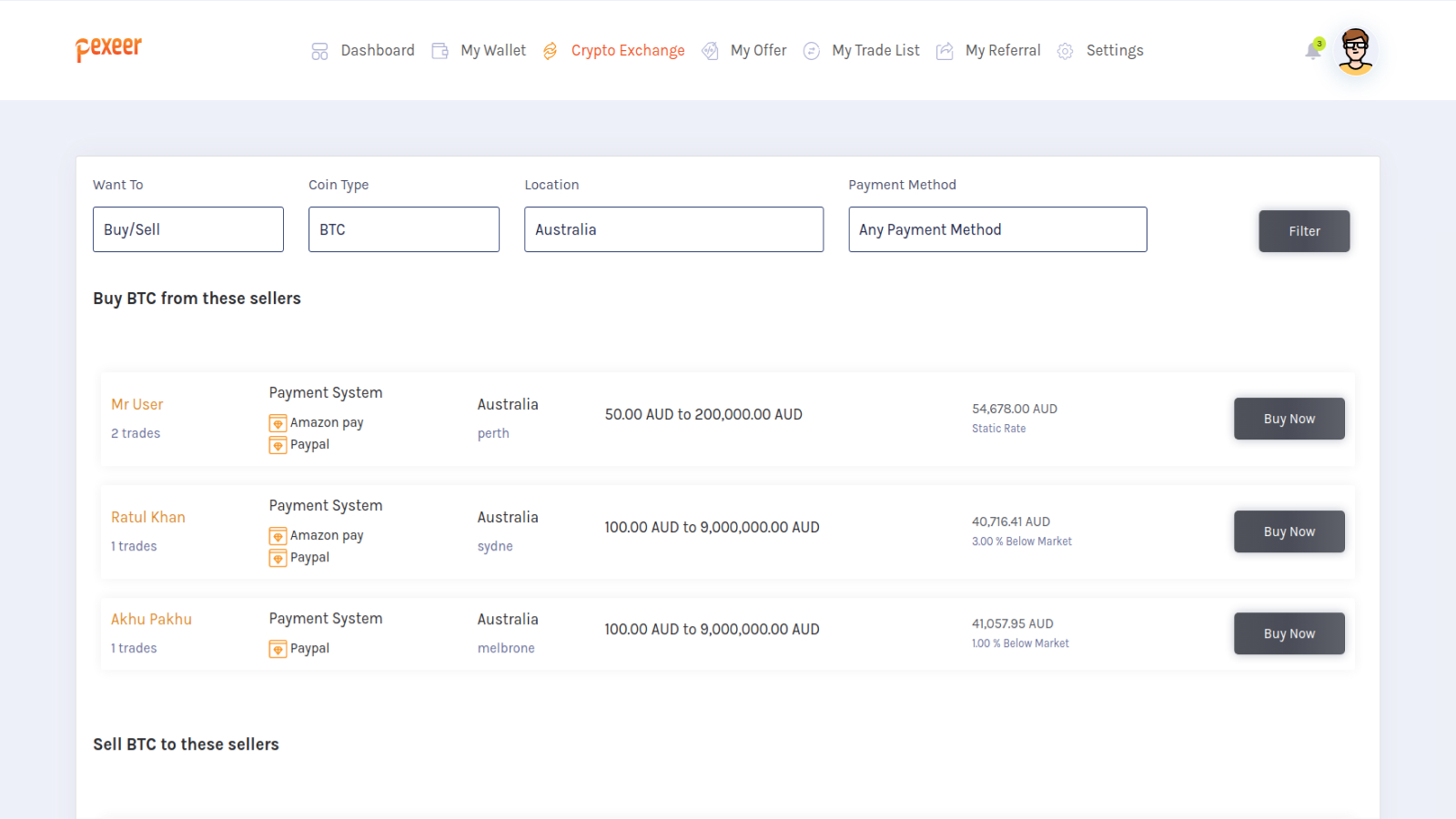A screenshot shows a CryPay feature dashboard for a crypto exchange. The interface, set against a gray background, includes multiple sections such as "My Wallet," "My Offer," "My Trade List," and "Referral Settings." Various buttons, including "Buy Now" and options for "Any Payment Method," are visible. A small avatar of a person is displayed with a white backdrop, contrasting against a larger gray background with a more prominent box. This appears to be part of a setup for managing payments. Additionally, terms like "BPC type" and "fundraiser for KubeKube" are mentioned, although specific instructions for making a payment are unclear from the screenshot.